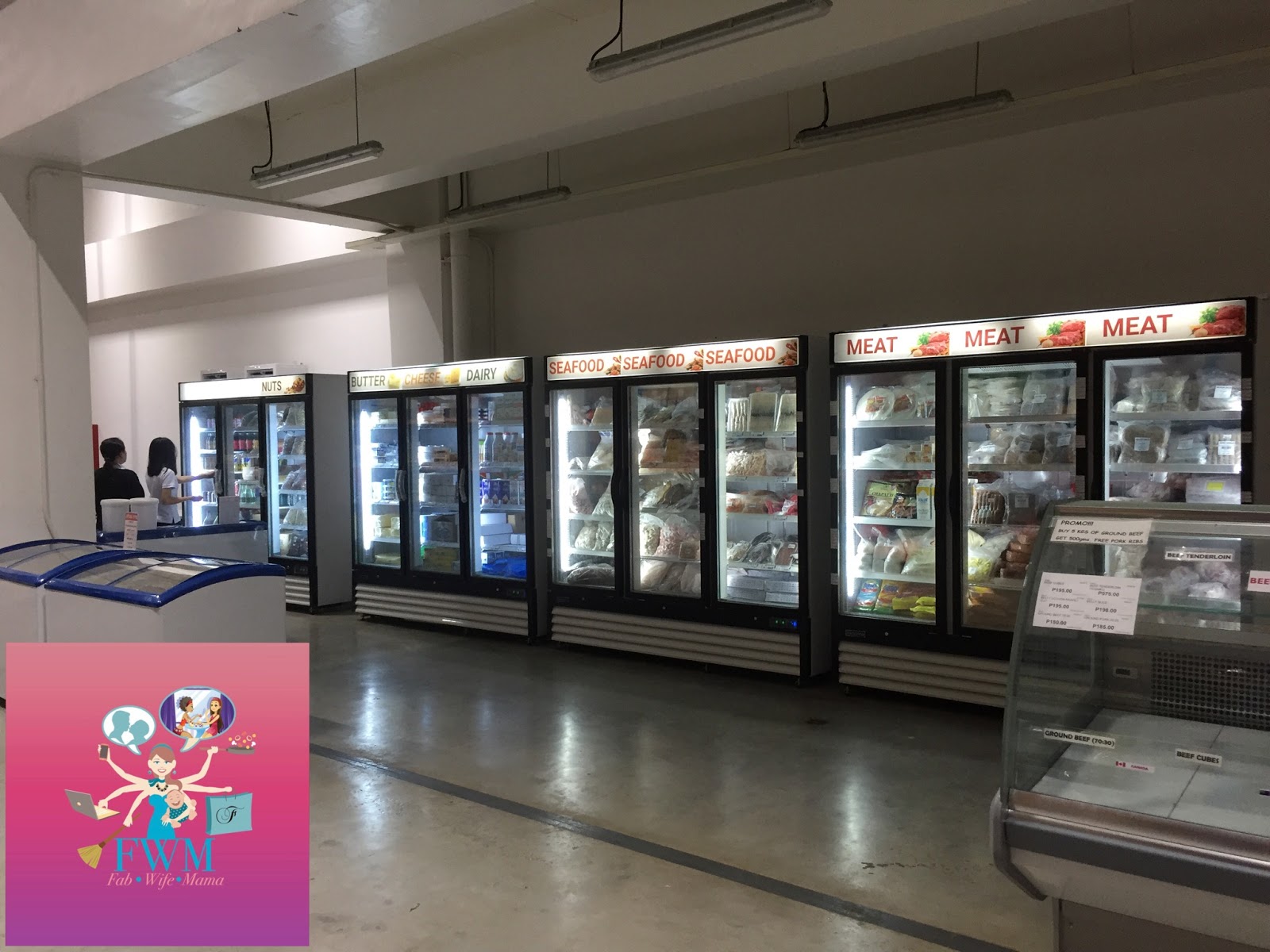The image depicts the interior of a well-lit eatery or restaurant, likely located in an Asian country. The walls in the background are pristine white, with several modern hanging lights providing ample illumination. Spanning from the far left to the right side of the image are walk-in coolers, resembling those found in grocery stores for storing frozen or refrigerated goods.

In the far left corner, two females are preparing to open one of these coolers. They both have long black hair; one is wearing a white shirt while the other is dressed in black.

The coolers have illuminated signs above them, indicating their contents. The cooler on the left is labeled "Butter and Dairy" and is adorned with corresponding images. The central cooler is marked "Seafood" repeatedly, featuring pictures of seafood items, while the cooler on the right displays "Meat" multiple times alongside an image signifying various types of meat.

On the bottom left-hand corner of the image, there is a large, pink graphic square created by a graphic artist. This artwork depicts a Caucasian woman with brown hair, possessing six arms, engaged in multiple activities. She holds a baby, works on a computer, cooks, and interacts with chat bubbles, illustrating her multitasking abilities. Below this graphic, the initials "FWM" are written in blue, and to the left of the square, there is a diagonal broomstick.

The combination of both grocery store elements and artistic graphics hints that the setting could potentially be an innovative store rather than a conventional restaurant.